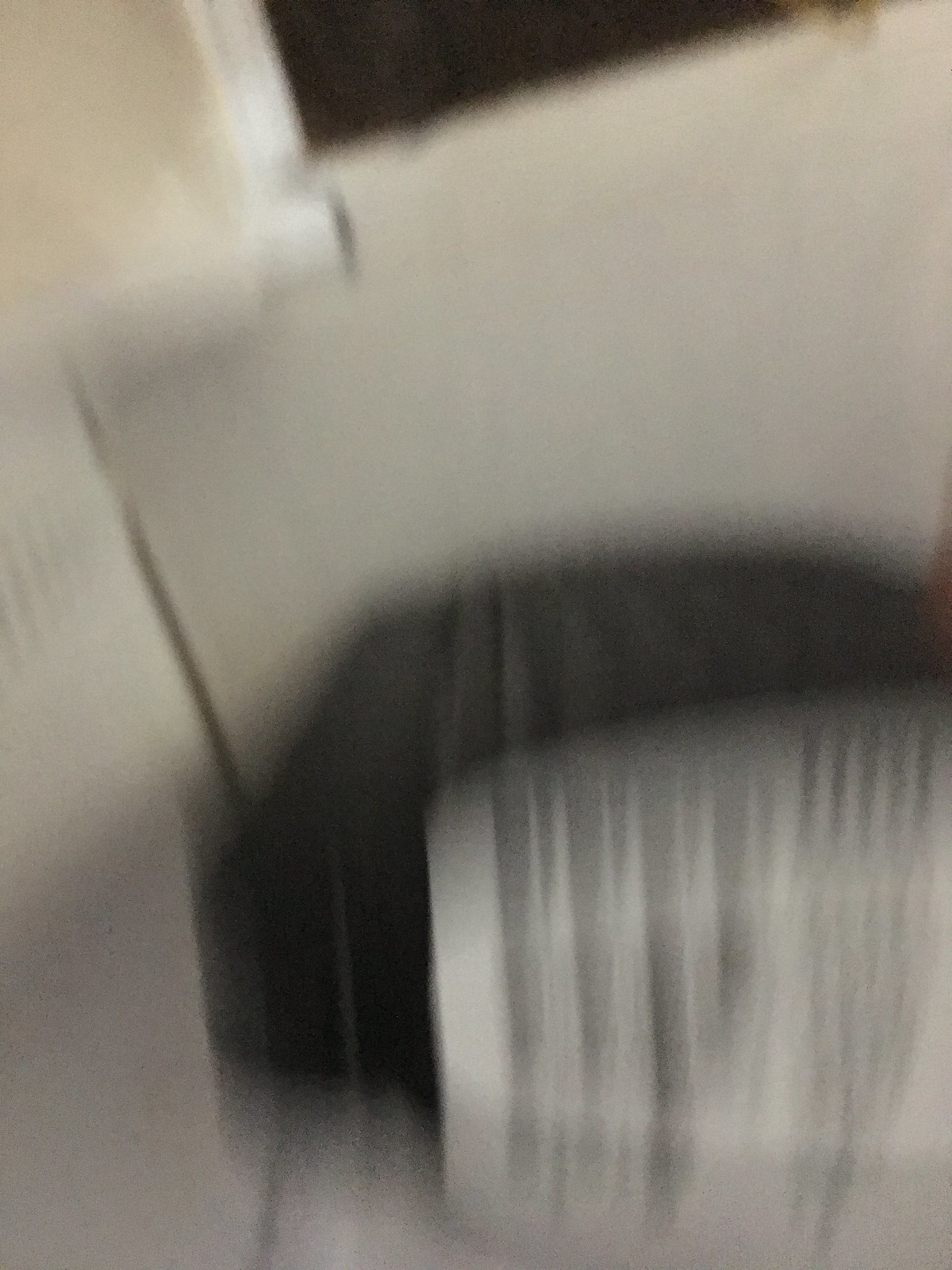In this photograph, the image is heavily blurred, likely due to camera movement or the motion of the objects being photographed. The scene appears to be set in a corner, with predominantly white surfaces dominating the background. The upper portion of the image features a dark area, creating a stark contrast against the lighter surroundings. Within the corner, two indistinct objects can be discerned. The object farther from the camera is a very dark grey, possibly black, while the object closer to the lens is white with darker stripes. Due to the severe distortion, it's challenging to accurately identify the objects or their shapes.